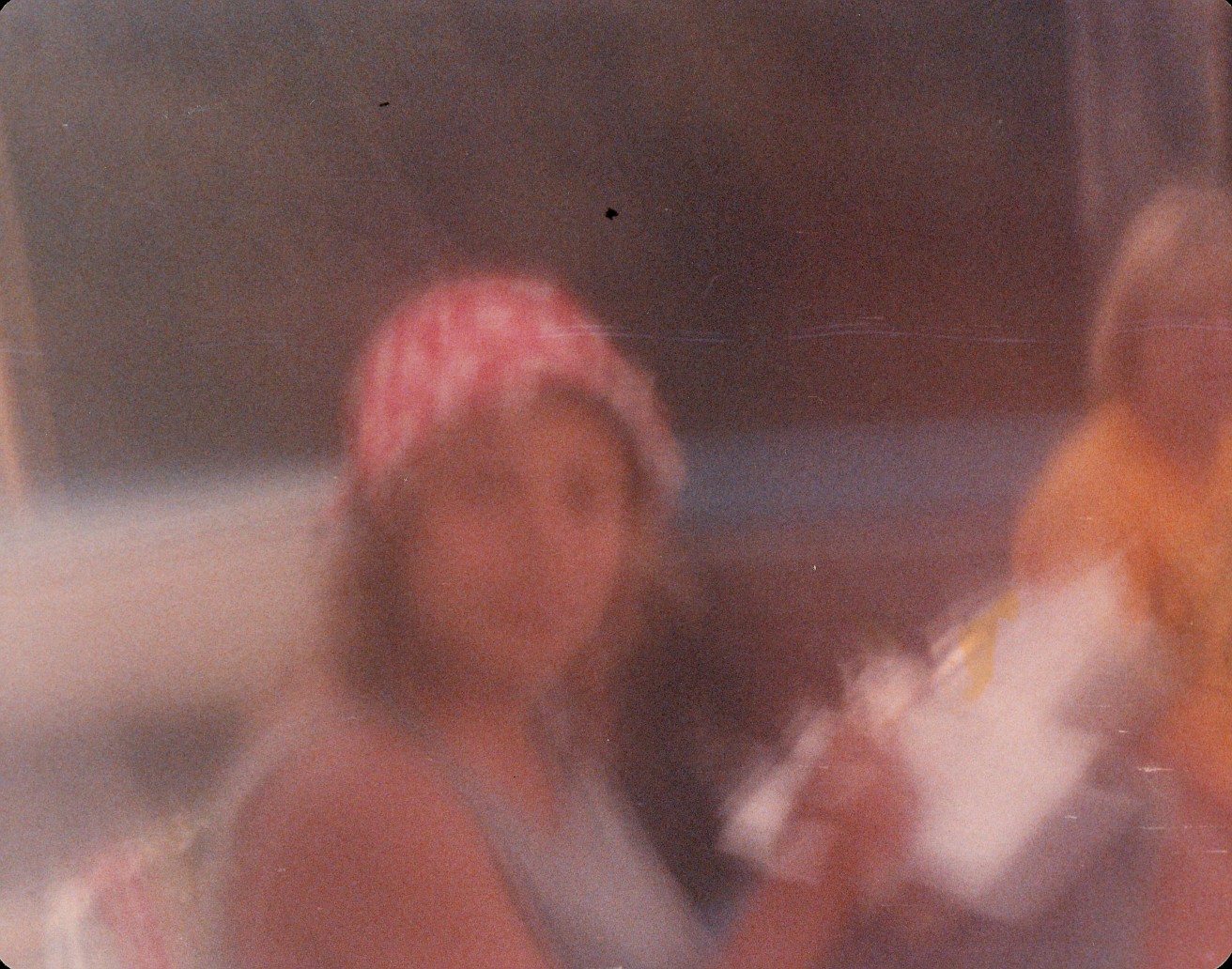This color photograph, though blurry, captures a tender domestic scene. In the foreground, a young girl with blonde hair, adorned in a red and white hat and a gray tank top, sits in a red and white striped chair. She holds what appears to be white paperwork in her hands, looking intently toward the camera. In the distance to the right, an older woman with chin-length blonde hair and possibly wearing glasses, is dressed in an orange t-shirt. She stands near a large window framed by a white sill, adding a touch of natural light to the scene. The juxtaposition of the girl’s focused expression and the background detail suggests a moment of quiet activity or contemplation.